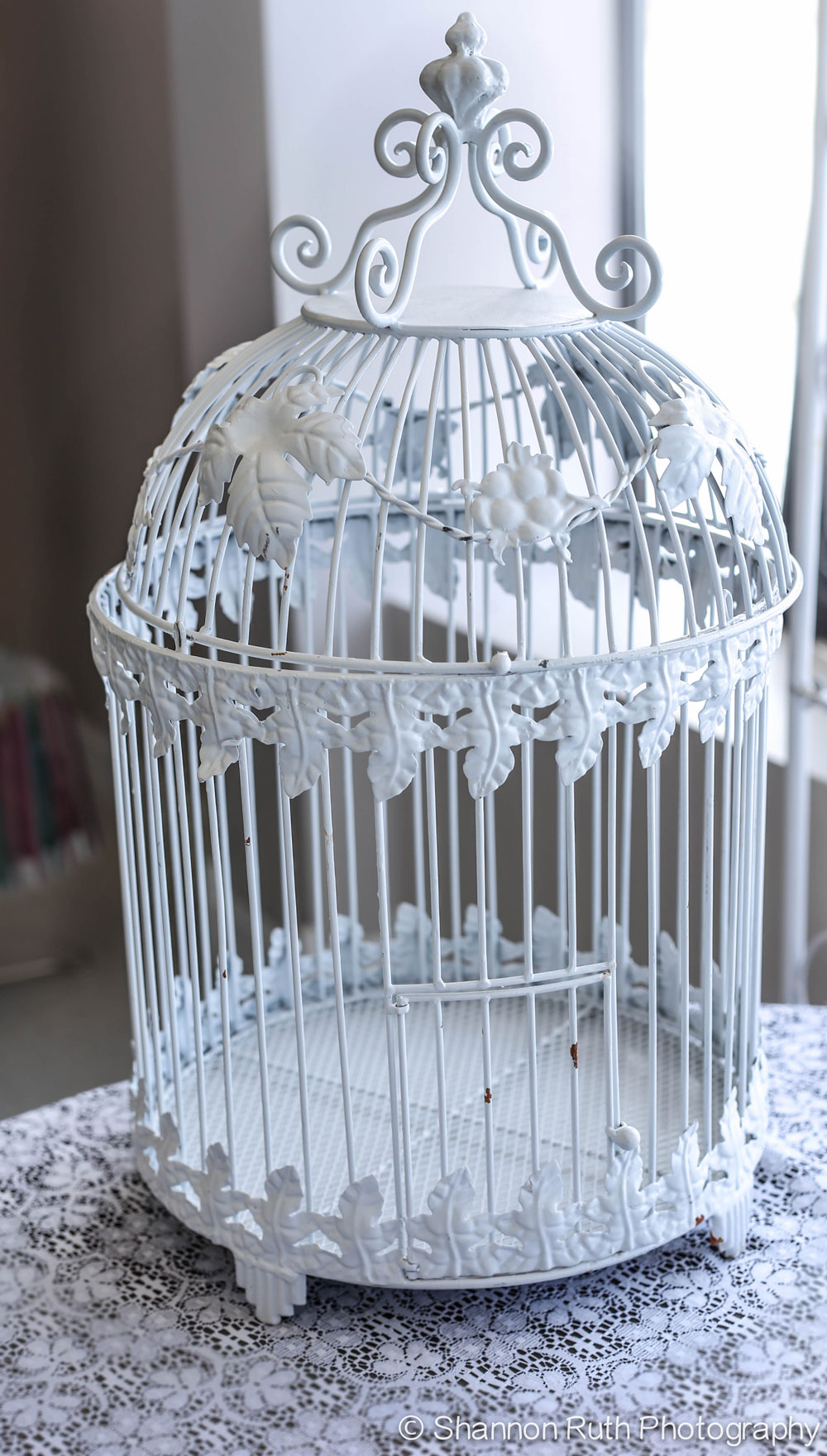The image showcases a vertically aligned, close-up photograph of an ornate, white birdcage. Measuring approximately one and a half to two feet tall, the birdcage, made up of delicate, thin white metal rods, sits elegantly on a table covered in a pristine white lace tablecloth. The round base sprouts thin rods that curve upward and converge at a circular rod, topped with a flat, circular lid. The lid features an upside-down arch design leading to a handle adorned with a diamond-shaped white knob, from which four delicate rods scroll down.

The birdcage, empty and closed, rests on small pedestal feet. Intricate designs, including floral patterns, leafy embellishments, and clusters of grapes, adorn its structure. At the very top, an ornate piece resembling a heart adds to the overall intricate design. Behind the birdcage, a window with an ambiguously blended and blurred background provides a subtle backdrop, complemented by a dark gray wall. The birdcage door faces the camera, and although the photograph is detailed, the photo credit in the lower right corner reads "Shannon Ruth Photography," difficult to make out against the white tablecloth.